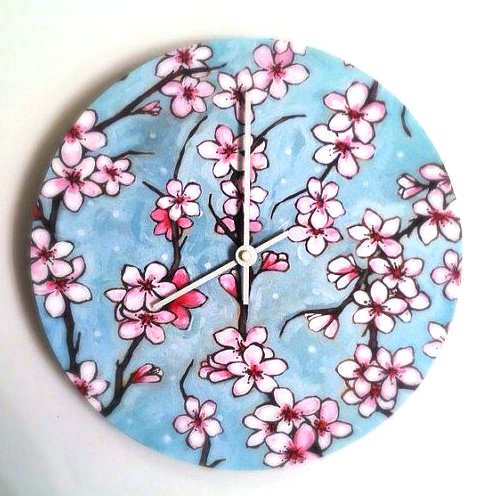The image depicts a detailed photo of a round, blue clock face set against a white wall. The clock face itself features a painted design with an array of pink cherry blossom flowers, each possessing at least five petals and dark pink stamens, along with slender brown branches that entwine their way across the background. Accentuating the floral theme, subtle white dots resembling snowflakes are scattered over the blue surface. Centrally located, two white clock hands are visible: a longer one pointing vertically upwards and a shorter one pointing towards the bottom left. The well-lit, white backdrop enhances the focus on the vibrant and intricate details of the clock's artistic design, creating a visually captivating and harmonious composition.